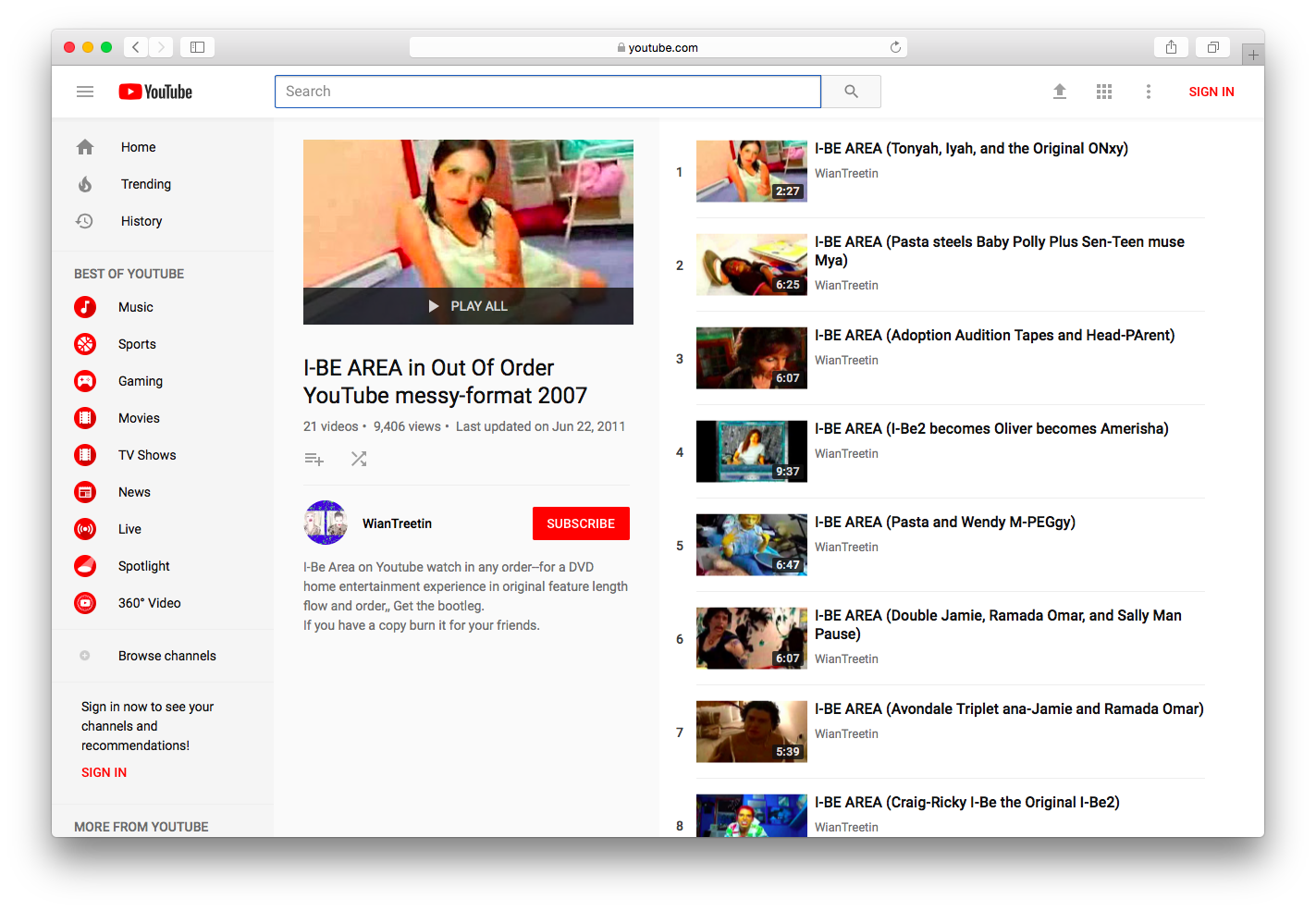Screenshot of a YouTube playlist page titled "I-BE Area" by the user WINTERTREATIN. The highlighted video currently selected is "I-BE Area in Out of Order YouTube Messy Format, 2007." 

The video just above it displays a woman lounging on a blue rug in a living room, adorned in yellowish lingerie. There is furniture visible behind her, enhancing the cozy and intimate setting.

On the right-hand side, the playlist is visible, showcasing a total of seven videos, each beginning with the title "I-BE Area" followed by additional descriptive content. On the left, the standard YouTube menu is presented, featuring options like Home, Trending, History, and Best of YouTube, among others.